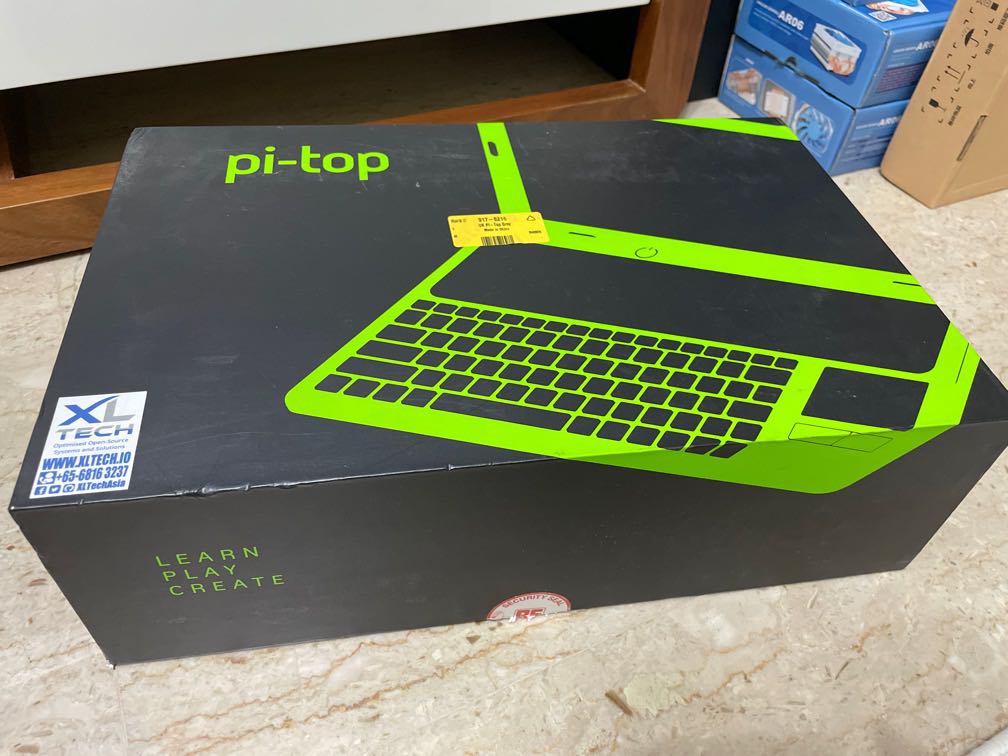A vibrant and sizable neon green box resembling a shoebox sits prominently in the image, designed to house a laptop branded as Pytop. The box features a catchy tagline that reads "Learn, Play, Create," emphasizing its educational and recreational potential. The bold, bright design of the packaging bears a striking resemblance to the characteristic colors of Xbox branding. A sticker located on the left-hand side of the box displays the name "XL Tech," hinting at a possible subsidiary or association, although the brand Pytop itself may not be widely recognized. The box has been carefully positioned for the photograph, suggesting a promotional intent, possibly to showcase the product's appeal or advertise it for sale.